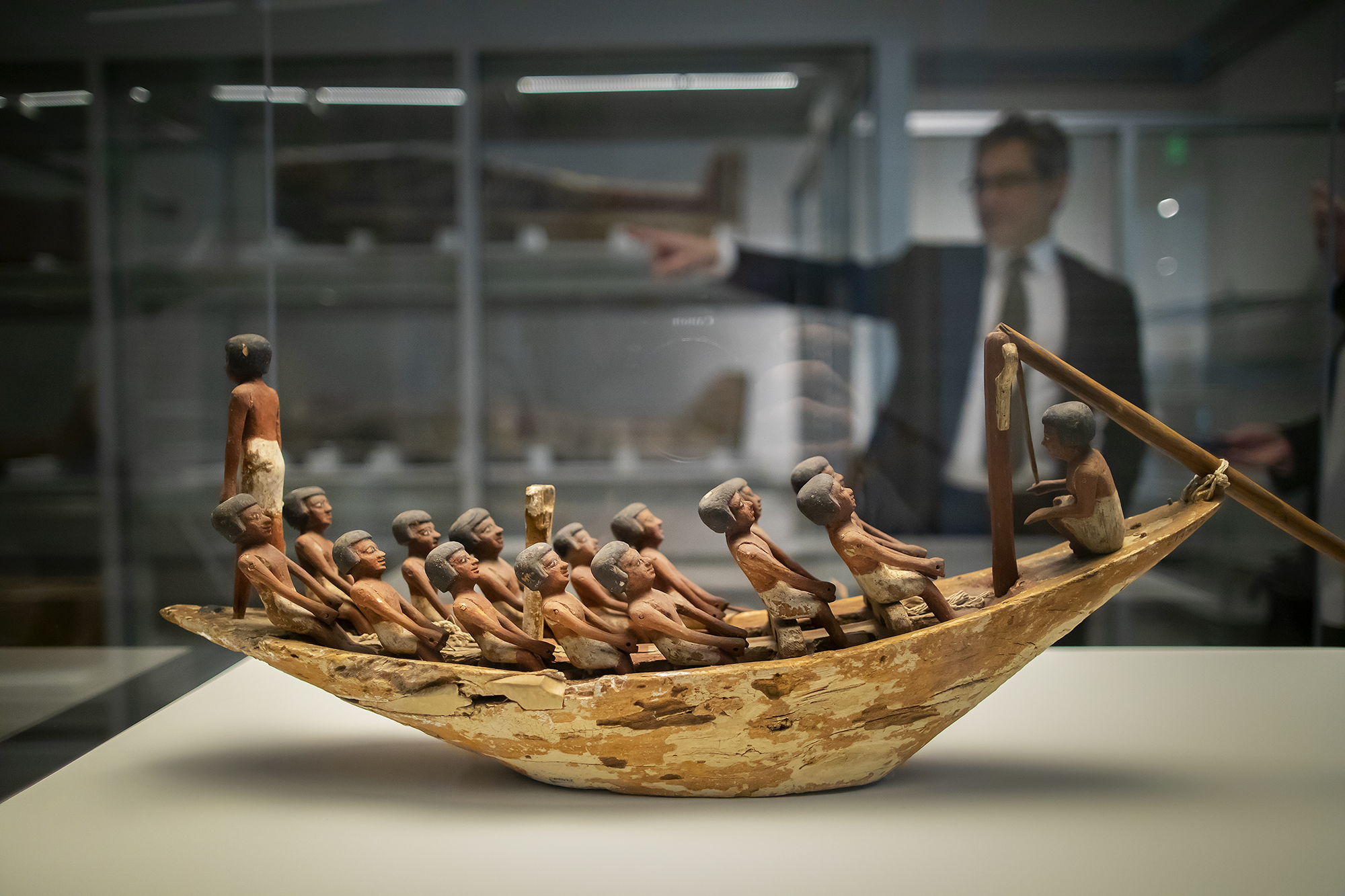This photograph captures an ancient Egyptian sculpture, likely made of pottery, depicting a boat with a pointed bow and stern, adorned with intricate details. The boat seats fourteen rowers, evenly distributed on both sides, all poised in a rowing motion, though their oars have long since disappeared, probably due to decay. A commanding figure sits at the prow, akin to a coxswain, directing the rowers, while another figure stands upright on the stern, overseeing the rear. The well-preserved artifact rests on a well-lit surface, perhaps within a museum's display area. The background is blurred, featuring shelves of other artifacts and a Caucasian man in a black jacket, white shirt, and dark tie, seen out of focus, gesticulating and pointing, highlighting the behind-the-scenes atmosphere of the setting.